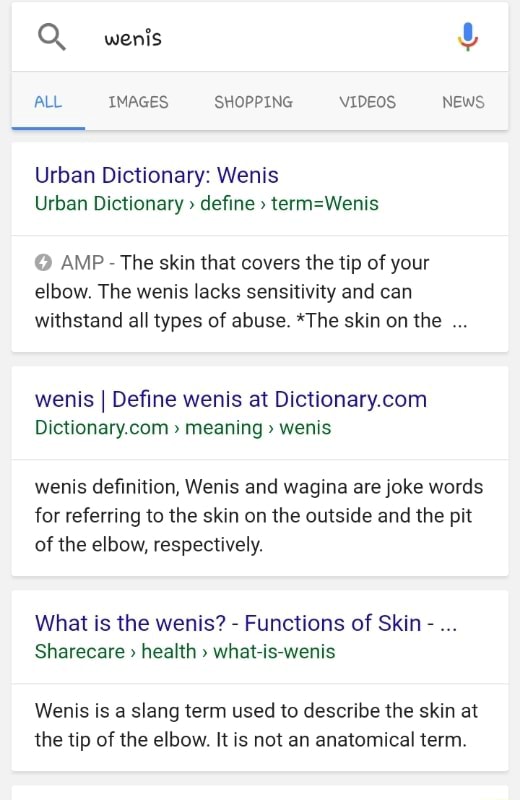The image captures a smartphone screen displaying a search results page. At the top of the screen, there is a recognizable search bar with a white background. On the left side of the search bar is a magnifying glass icon, and next to it, in bold black lettering, is the word "we-ness." On the right side of the search bar, there is a blue microphone icon, indicating voice search capability.

Below the search bar, there is a horizontal row of five interactive options in all capital letters. The first option, "ALL," is highlighted in blue and underlined, indicating it is the current selection. The other options are labeled in gray capital letters: "IMAGES," "SHOPPING," "VIDEOS," and "NEWS," suggesting alternative types of search results available.

The content below the navigation options is populated with search results related to "we-ness." The first result is displayed prominently in bolded navy blue text: "Urban Dictionary: we-ness." Underneath, in green text, it reads, "urban dictionary defined term = we-ness," providing further context. This entry includes an accompanying description: "The skin that covers the tip of your elbow. The we-ness lacks sensitivity and can withstand all types of abuse." There is a gray circle containing a lightning bolt icon to the left of this description, indicating an Accelerated Mobile Page (AMP) feature designed for faster loading. Below the partial description, three dots suggest additional information is available if the user taps on it.

Following this primary definition, the page continues with more entries and definitions related to the term "we-ness."